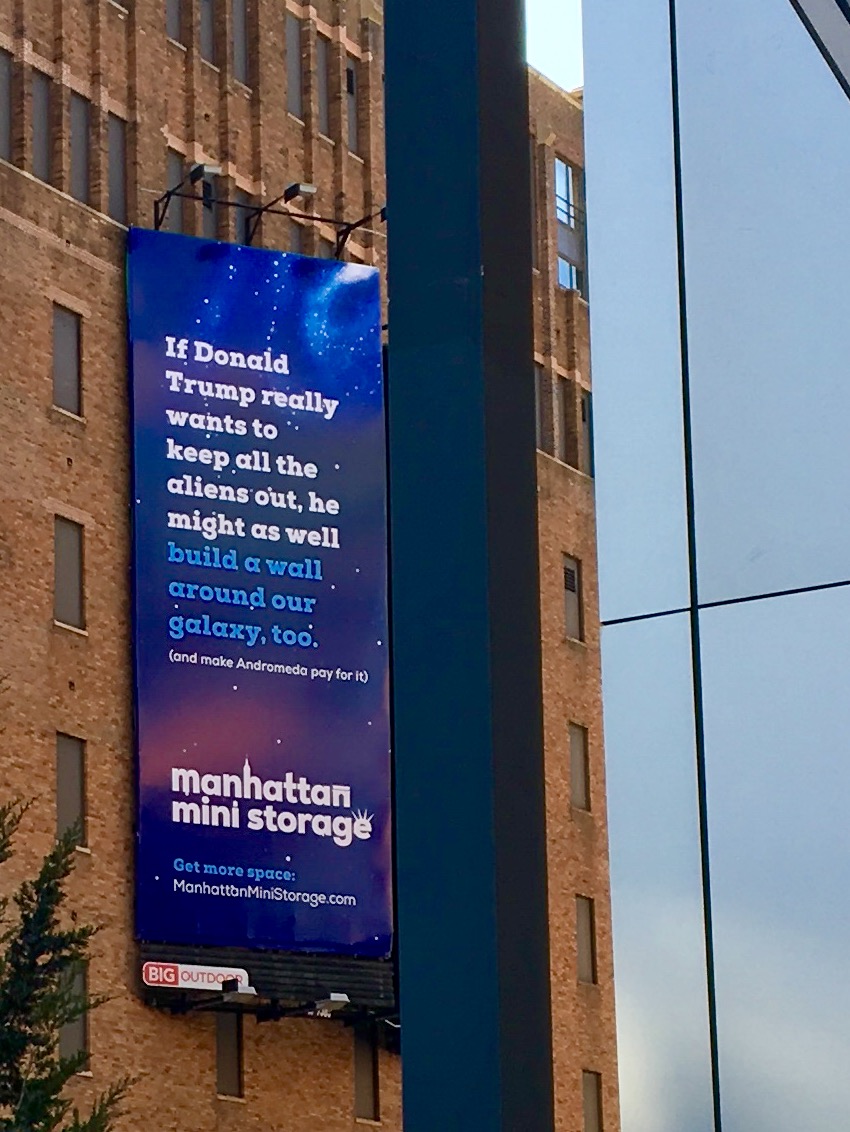This daytime photograph captures a vibrant street-level view of a large rectangular billboard mounted on black metal supports above a tall brown brick building, which spans from the bottom left to about two-thirds of the frame. The building features a series of windows, some boarded up, and a green tree partially obscuring the lowest window on the left side. The billboard itself has a striking navy blue and pink galaxy-like background, adorned with stars, and displays the humorous message: "If Donald Trump really wants to keep all the aliens out, he might as well build a wall around our galaxy too. And make Andromeda pay for it." Below this, it advertises "Manhattan Mini Storage" with the slogan "get more space" and a website address in white at the bottom. The sign is contrasted against a small sliver of blue sky in the upper left corner, while more brick buildings occupy the right side of the frame, connected by a large column with a blue banner about Donald Trump, aliens, and building a wall.